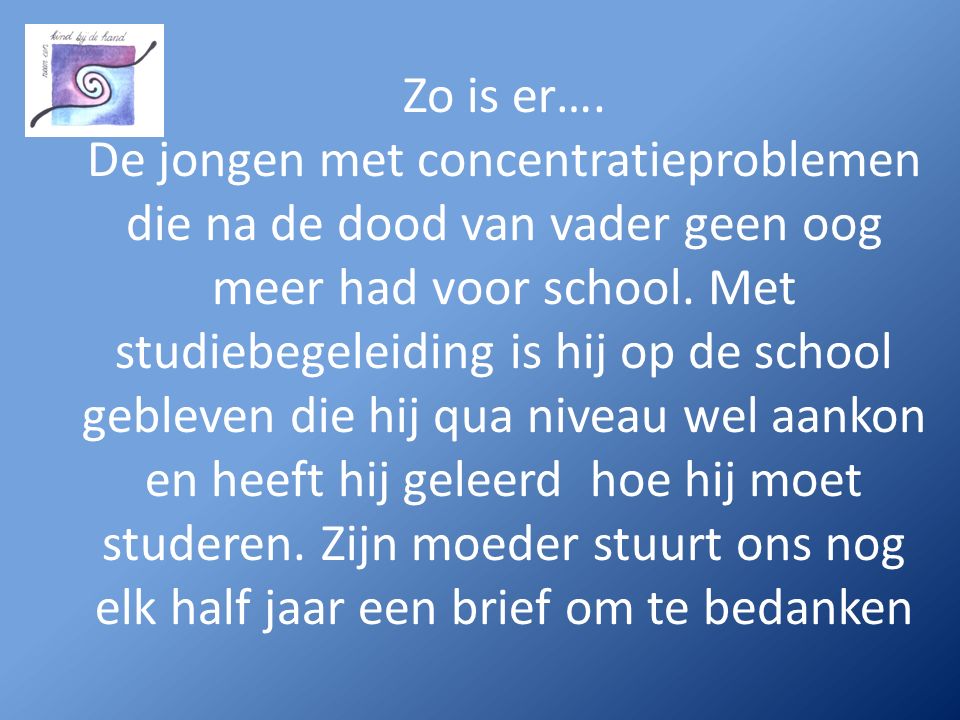This image features predominantly white text on a blue background, which transitions from a darker blue in the bottom right corner to a lighter blue towards the top right. Dominating the majority of the image, the text appears to be in Dutch. In the top right corner, there is a small logo comprised of purple and blue hues with a black spiral at its center. The image highlights various shades of blue, and includes an intricate design element in the form of a logo or stamp with words arranged in a spiral pattern, adding to the overall composition.